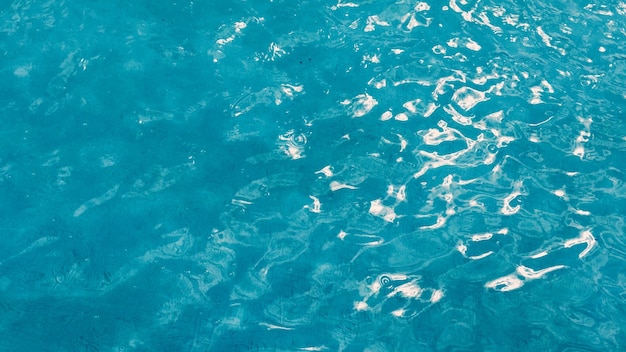The photograph is a full-color, horizontally rectangular image capturing the view of blue water from above, with no discernible background or borders. The water, likely from a pool, is very clean and varies in hues from darker to lighter blues, with visible ripples and small waves playing across the surface. The sunlight hits certain parts of the water, creating sparkling white areas and adding a refractive quality to the scene. The left side of the image appears slightly darker with less light reflection, while the right side is brighter and shows more pronounced rippling and light refraction. The bottom of the pool, tinted an aqua bluish-green, subtly influences the overall coloration of the water.